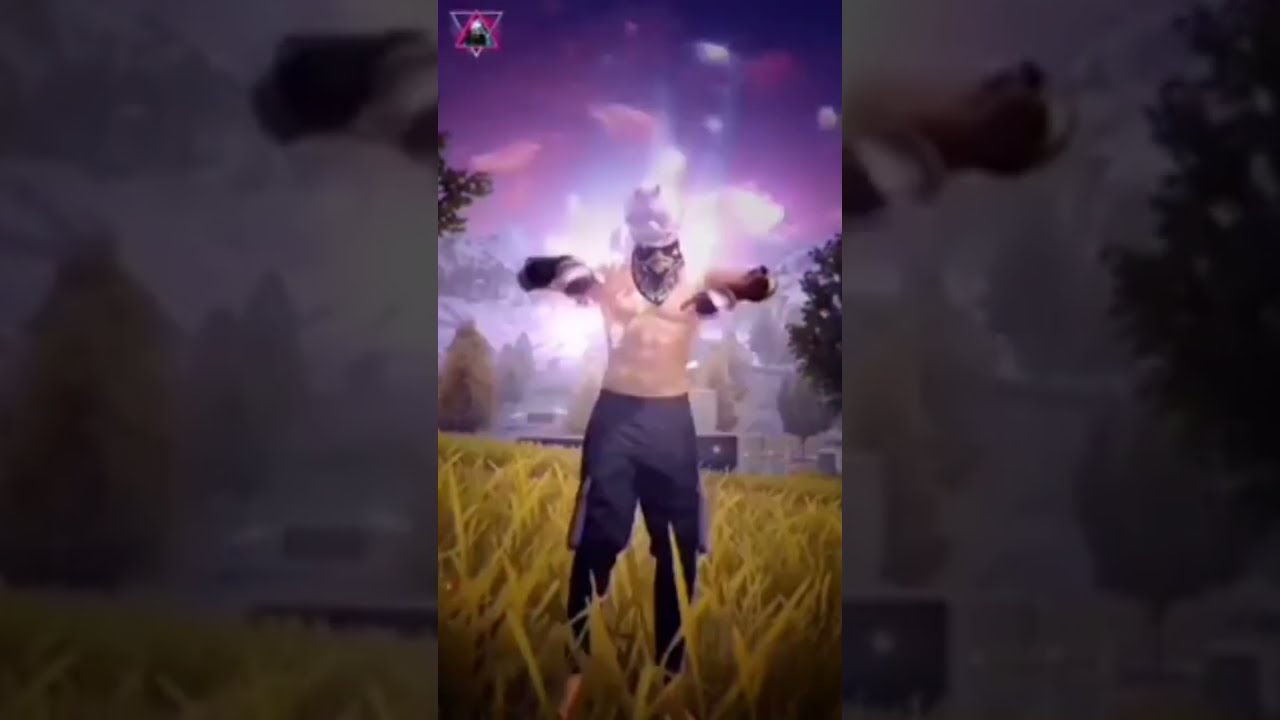In this digitally created image, potentially from a video game or fantasy animation, a character stands in the center of a knee-high golden wheat field under a purple-blue sky. The character is shirtless and has white skin, wearing black shorts, black leggings, dark gauntlets with extended wrist guards, and white wrappings around their hands. They have a striking crow-like head featuring a pronounced beak and dark eyes, suggesting they are wearing a bird mask. Perched atop the mask is a small, ambiguous white creature, adding to the surreal nature of the scene. The background reveals a combination of green trees, possibly snow-capped mountains, and a distant city under a sky illuminated by white bursts of light. The overall setting is enveloped in a twilight ambiance, hinting at a fantastical or otherworldly environment.